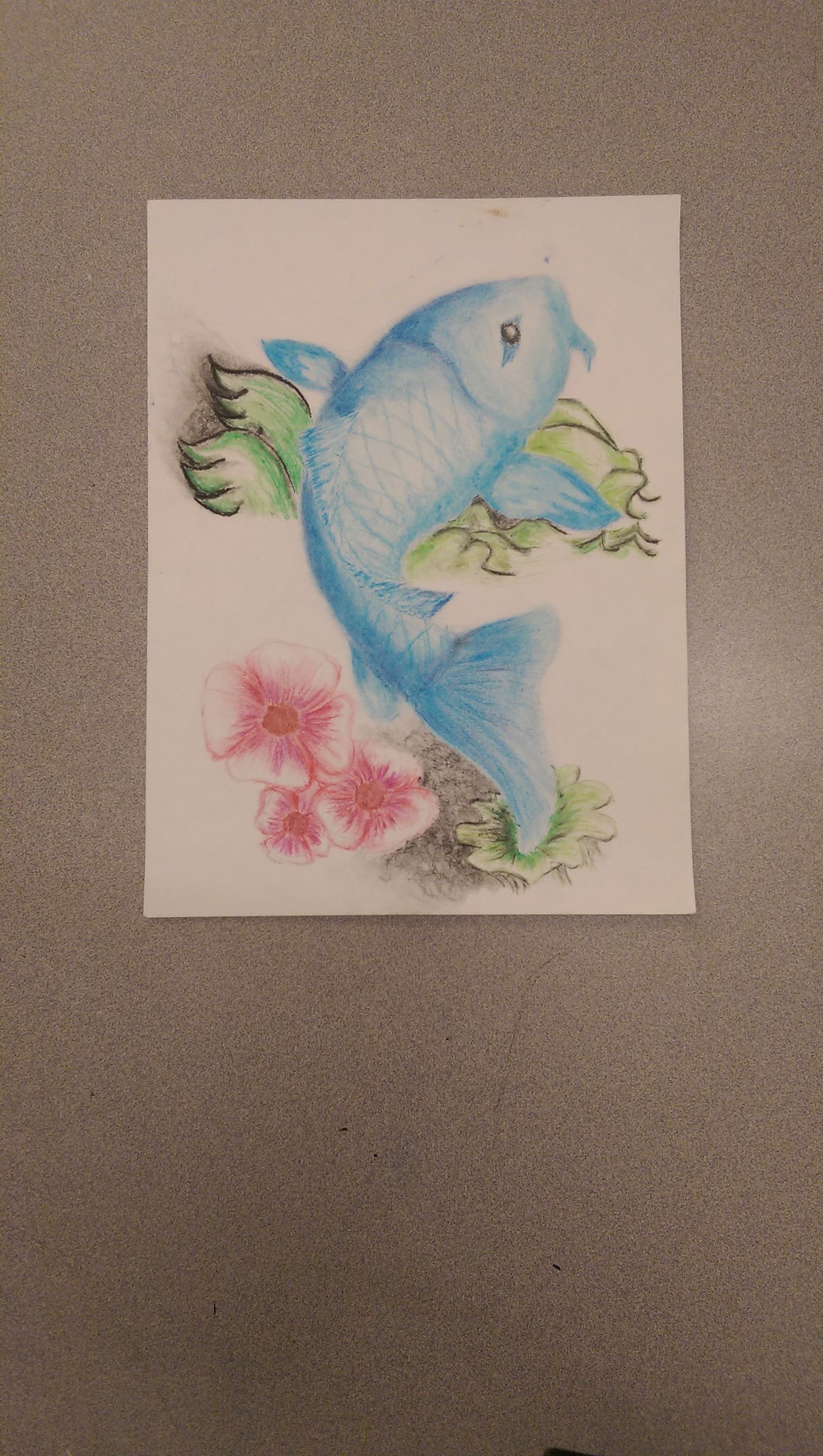The image depicts an intricate, hand-drawn painting of a blue fish, resembling a koi or betta fish, positioned against a gray, textured background, possibly resembling concrete or stucco. The fish features vibrant shades of blue, transitioning to white around its eyes and complemented by hints of green along its body. The fish is oriented with its head facing up and to the right, mouth open, and its tail flowing towards the bottom left. Surrounding the fish are various illustrations of greenery, likely intended to represent aquatic plants or flowers, adding depth to the scene. Below the fish, there are three white and pink flowers, each consisting of four petals that turn more pink towards the center, and featuring reddish or orangish centers. The entire illustration is executed on a white piece of printer paper that sits on the gray surface, potentially on a table. A minor crack can be seen on the background surface, adding a touch of texture to the scene.